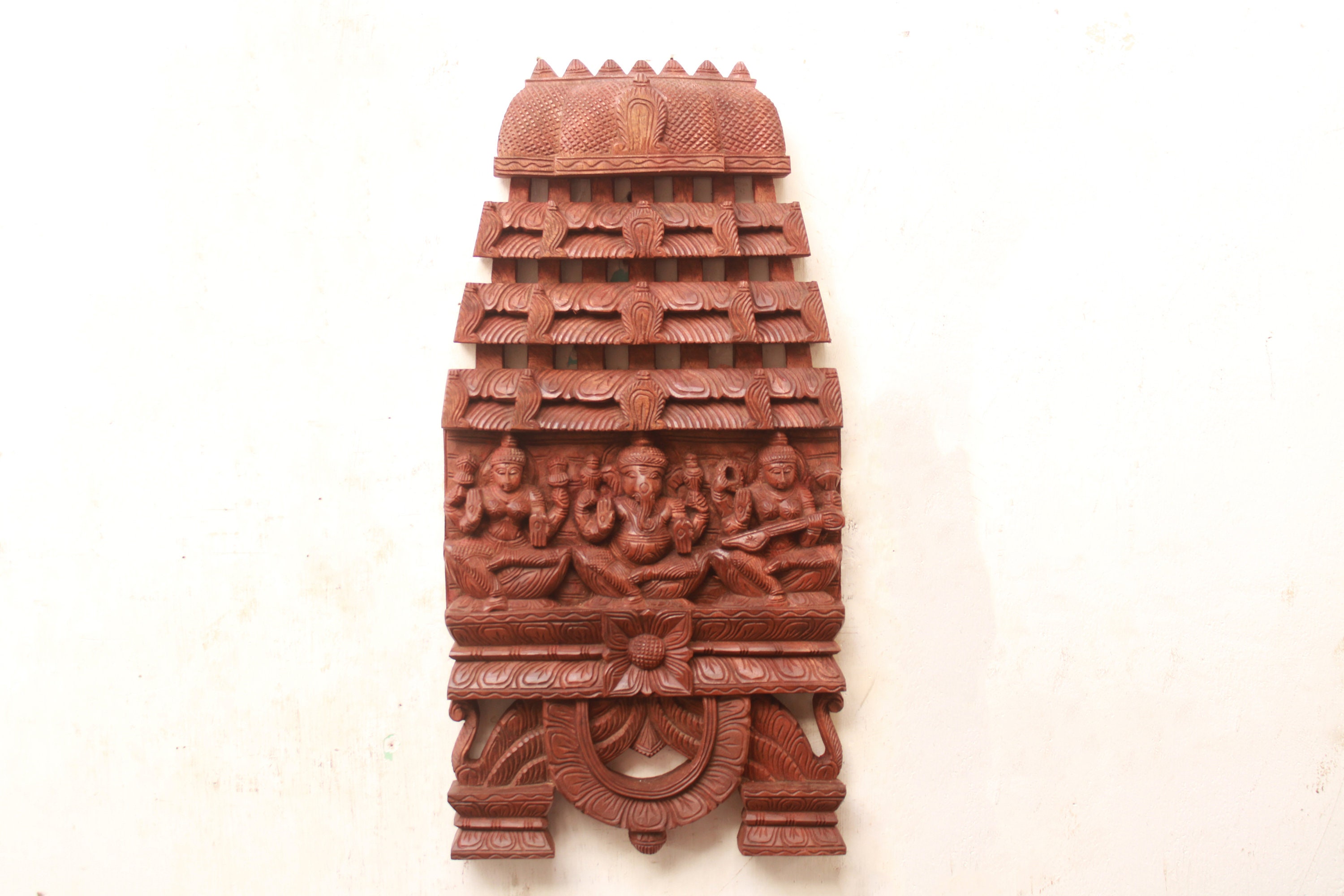The photograph captures an intricately detailed, ornamental wall sculpture, likely of Indian or Buddhist origin. The background is an off-white wall, which makes the red clay-colored sculpture stand out distinctly. The sculpture itself evokes the elegance of religious decor often associated with Indian temples. The central feature of the wall art is a floral pattern, carved meticulously into the material. Beneath this, three figures, possibly deities or worshippers, are depicted in a cross-legged sitting position, each holding musical instruments and adorned with headdresses. They are arranged beneath a three-tiered wave-patterned wood paneling, which further enhances the piece’s intricate design. The sculpture ascends into a tiered, temple-like roof structure with triangular stipples and spikes on top, giving it a striking, almost dome-like appearance. The entire piece, with its ornate patterns and religious iconography, appears to be hanging on the wall, skillfully blending artistry with cultural reverence.